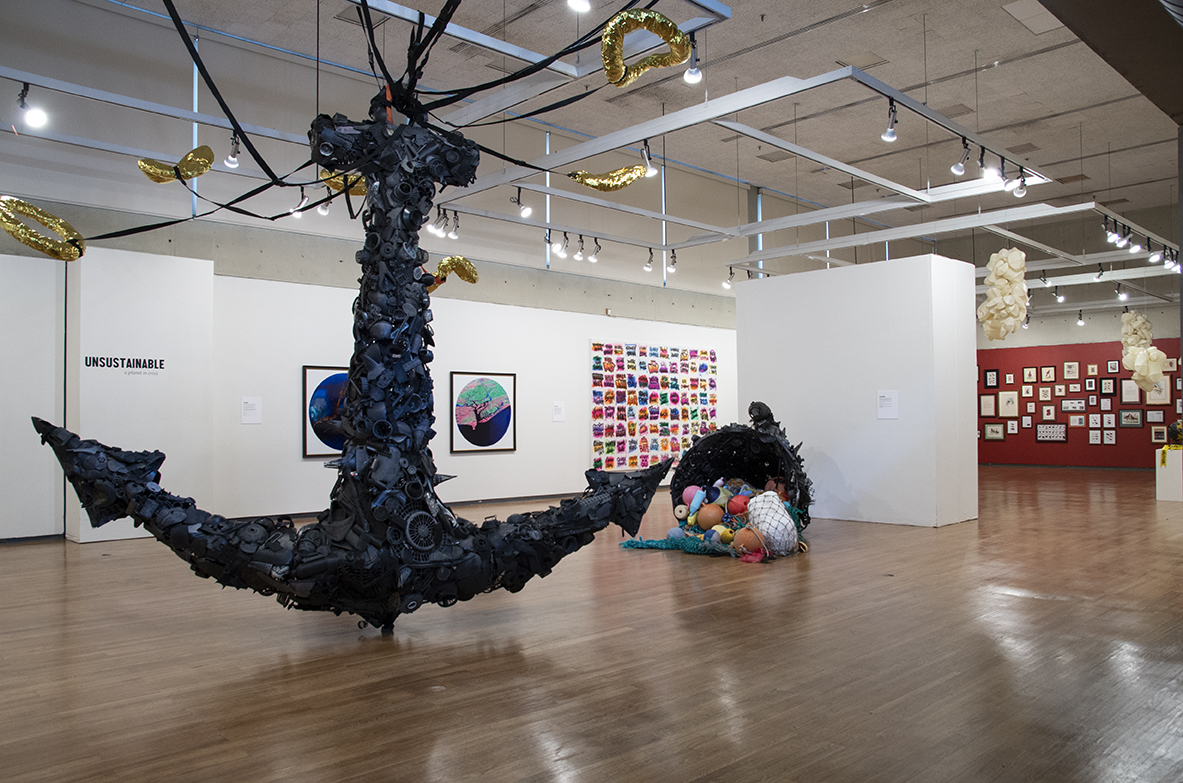In this image taken inside an art gallery, a large, intricately constructed anchor dominates the center, suspended from the white ceiling with sturdy lines. The anchor is made from a variety of reclaimed plastic and metal parts, including old camera lenses, fans, cans, and hubcaps, creating a visually captivating piece resembling an amalgam of junk. Beside the anchor, a black basket—also crafted from similar reclaimed materials—has its contents, which look like toys and eggs, spilled onto the shiny, light brown wooden floor.

The gallery space features white walls adorned with various artworks. To the left of the anchor, the word "unsustainable" is prominently displayed on the white wall. On the far right, a burgundy wall showcases several framed art pieces. Additionally, the left wall features paintings of circles in green and blue, with one artwork being entirely blue. This detailed, eclectic setup captures the essence of modern, abstract art within the gallery's vibrant atmosphere.